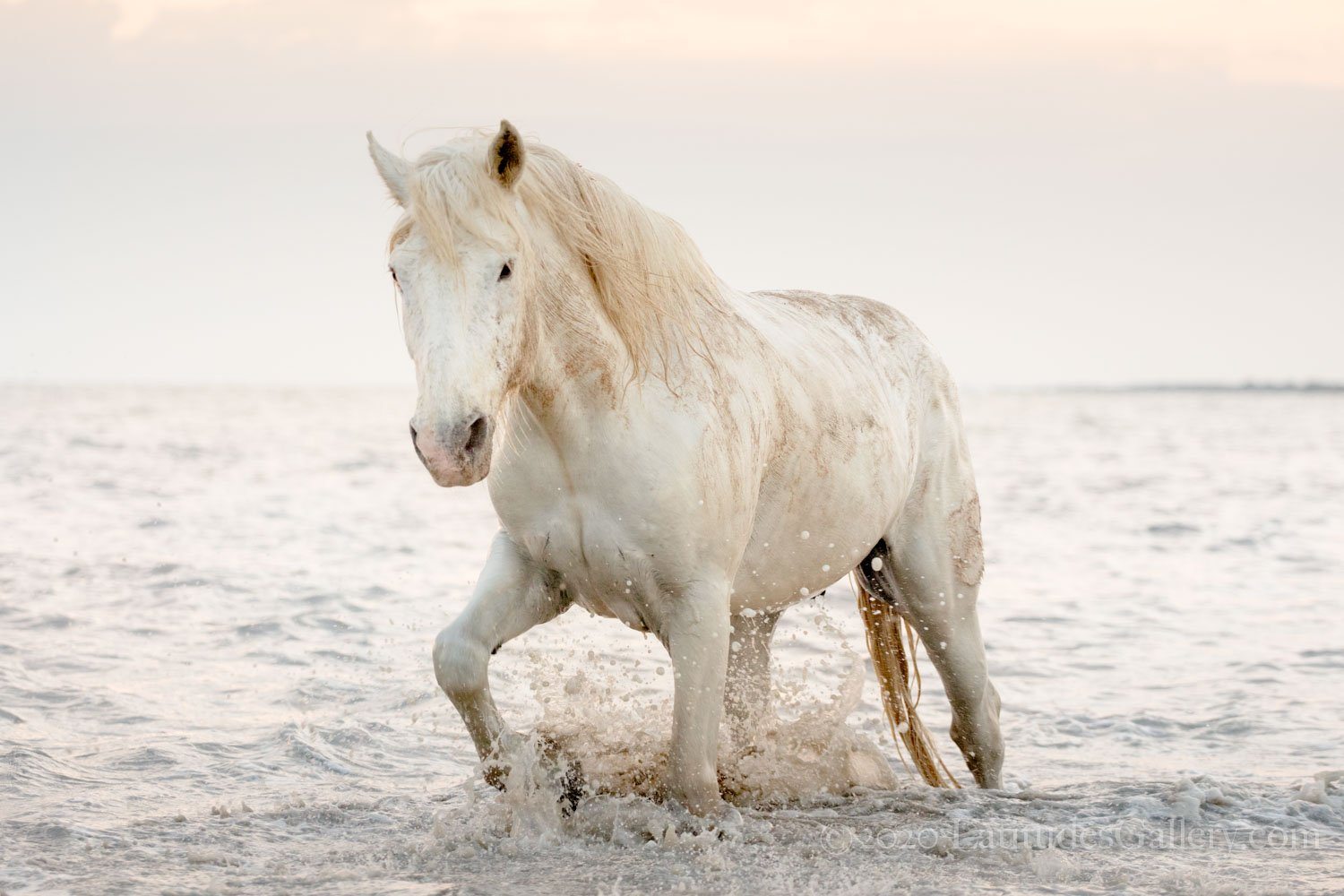A striking photograph captures a large, wild white horse with a speckled coat of brownish-tan spots, running through what appears to be an ocean or lake near the beach. The water around the horse is splashing violently as it lifts its front legs, with droplets cascading down its wet tail and body. The horse is facing the camera, its black eyes and nostrils prominent against its otherwise white face, with dark inner ears contrasting the white outer fur. The scenery is suffused with a whitish cast, with a sky and ocean that appear washed out. The background is tinged with subtle pinks, violets, and touches of blue, enhancing the surreal and serene quality of the image. A watermark at the lower right corner indicates the source as 2020latitudesgallery.com. The overall ambiance is one of ethereal beauty, capturing the essence of the horse's power and grace amidst a tranquil, almost dreamlike seascape.